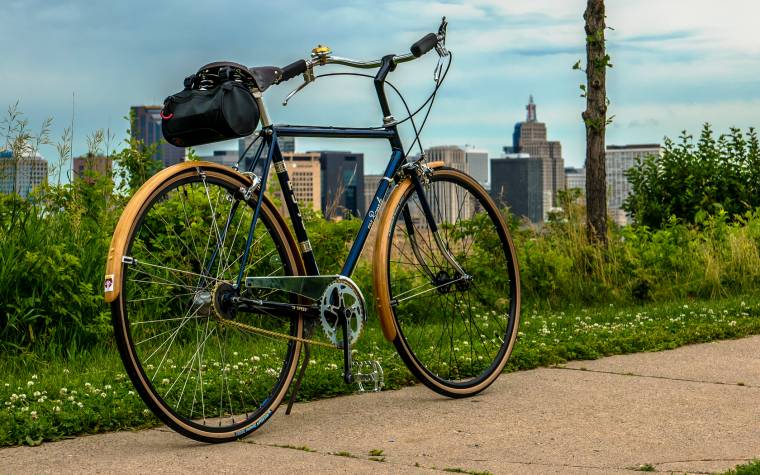The image showcases a lightweight, navy blue bicycle parked slightly left of center on a gray sidewalk, with the kickstand down. The bike features gold-colored fenders over both tires, which have black exteriors and gold-colored rims with thin spokes. The rear sprocket is gold, while the one near the pedals is silver, connected by a gold-colored chain. The bicycle's footrests include a black arm and silver footrest. It has a black seat with a black backing and a small black bag hanging behind it. The chrome handlebars boast black hand grips and chrome brake levers with black wires. Notably, a gold bell can be seen on the left handlebar.

Surrounding the bicycle, the sidewalk displays patches of green vegetation peeking through the cracks. Directly behind the bike is a mixture of green weeds, some with yellow flowers, and a large tree trunk with branches and leaves. The background reveals a city skyline filled with tall, gray, black, and brown skyscrapers against a hazy sky of gray and white clouds, with a hint of blue.